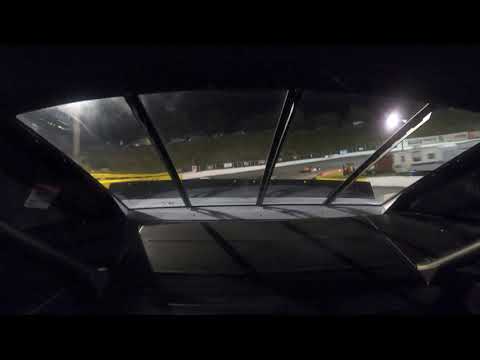The photograph captures a nighttime scene, taken from inside a vehicle's cockpit, with an expansive view through a large, curved four-pane window reminiscent of a car's windshield. The interior of the vehicle is cast in shadow, accentuating its black finish, and features long, thin metal arms extending diagonally. Through the window, the dark sky is punctuated by bright stadium lights on both the left and right sides. Outside, the curved structure of an empty stadium is visible, dotted with sponsor signs on fences, and the view reveals a racecourse with a few cars navigating the track. To the right, white trailers, possibly for sports players or maintenance workers, stand against the dark backdrop, adding to the scene’s depth. Curved stands and distinct sections are illuminated by street lamps, creating a vivid contrast with the night.